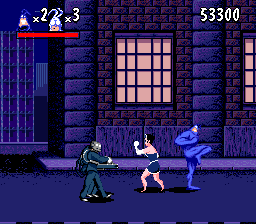This screenshot is from the classic SNES video game, "The Tick." At the center of the frame stands a villain dressed in navy clothes, holding a gun aimed at a white woman who is dressed in a blue tank top, blue shorts, and white gloves. She is positioned as if ready to fight. Positioned to the right is the main character, The Tick, a superhero clad in a full blue costume, with one leg raised as if he is about to deliver a kick. They are all set against the backdrop of a brick building on a nocturnal street. In the upper left corner of the screen, the players' remaining lives are displayed as '2' and '3' respectively, accompanied by a health bar. Meanwhile, the upper right corner showcases the score, reading 53,300.